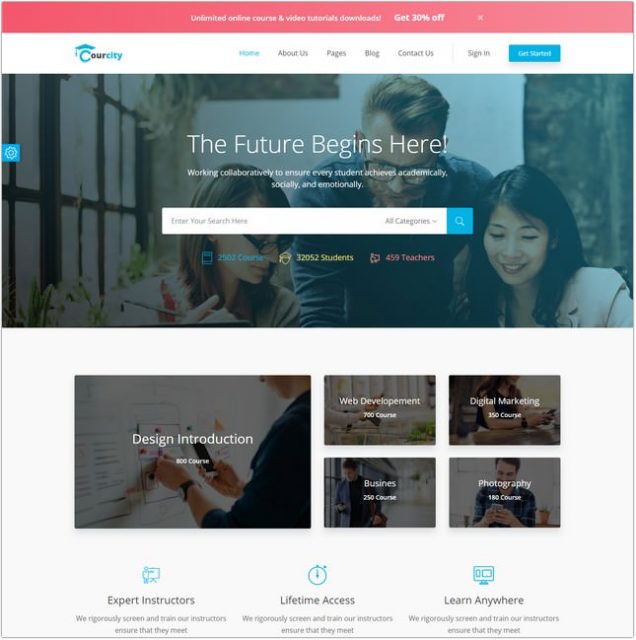In this image, we have a detailed view of a webpage designed for an educational platform. The top left corner displays a security icon, indicating a secure and protected site. Prominently featured is the logo for "Tower City." The website header showcases a promotional message: "Unlimited Online Courses and Video Tutorials. Downloads. Get 30% Off."

Navigational links are clearly visible, including "Home," "About Us," "Pages," "Blog," "Contact Us," "Sign In," and "Get Started." Additionally, the site carries the inspirational slogan, "The Future Begins Here," highlighting its mission of "working collaboratively to ensure every student achieves academically, socially, and emotionally."

A search bar is available with an option to search across "All Categories." Key metrics are prominently displayed, showing 2,502 courses, 2,052 students, and 459 teachers. Course categories are broken down as follows: Design Introduction with 800 courses, Web Development with 700 courses, Digital Marketing with 250 courses, Business with 250 courses, and Photography with 180 courses.

The site emphasizes the quality of their instruction with a section on "Expert Instructors," noting that the platform "regularly screens and trains our instructors to ensure they meet our high standards."

The color scheme of the webpage includes a combination of red, blue, gray, and white, creating a visually cohesive and inviting environment for users.